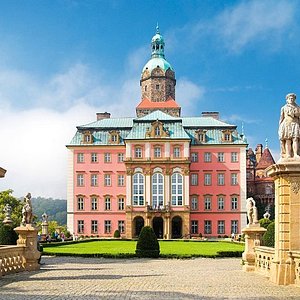The image depicts a prominent building resembling a European castle or a historic Ivy League campus structure, possibly reminiscent of Harvard. The building itself stands at six stories high, featuring a distinctive green tin roof and a notable watchtower topped with a small blue tower. This mansion-like structure is made of pinkish bricks and showcases three arched windows above three arch entries.

In front of the building, there is an expansive circular drive-through encircling a lush green courtyard with meticulously manicured grass. Two areas of yellowish stonework flank the entrance, each adorned with statues of people. Additionally, the ground around the structure is a mixture of neatly laid concrete and brick pavement with grayish white dirt. A statue of a woman in gray is prominently positioned atop one of the stone structures, adding to the grandeur of the scene.

The background features additional buildings and a landscape filled with numerous trees, all set under a vast blue sky dotted with clouds. The overall ambiance suggests an academic or historically significant setting, characterized by its architectural elegance and well-maintained surroundings.